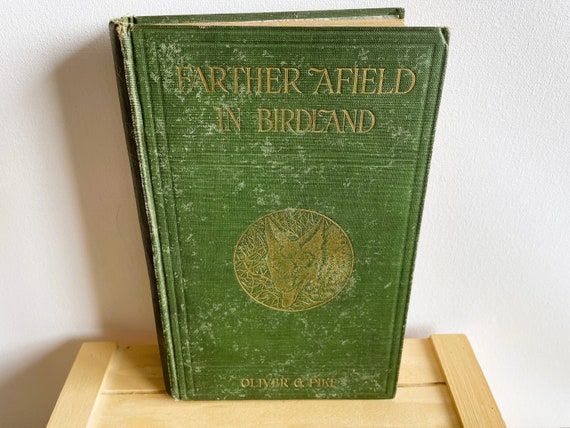This photograph captures a very old, worn leather-bound book prominently displayed on a small beige stand. The book, titled "Father of Field and Birdland" by Oliver and Pike, is a dark green color with frayed edges, showcasing its age. Its cover is adorned with gold lettering and features a large gold medallion, which bears an intricate but faded image that most likely depicts a wolf amid branches, emphasizing a nature theme. The book's condition, with its thick, compressed paper and evident wear, highlights its vintage nature. The setting is simple, with the book positioned against a light gray or white wall, either on a wooden table or shelf, enhancing the focus on this distinguished, historical artifact.